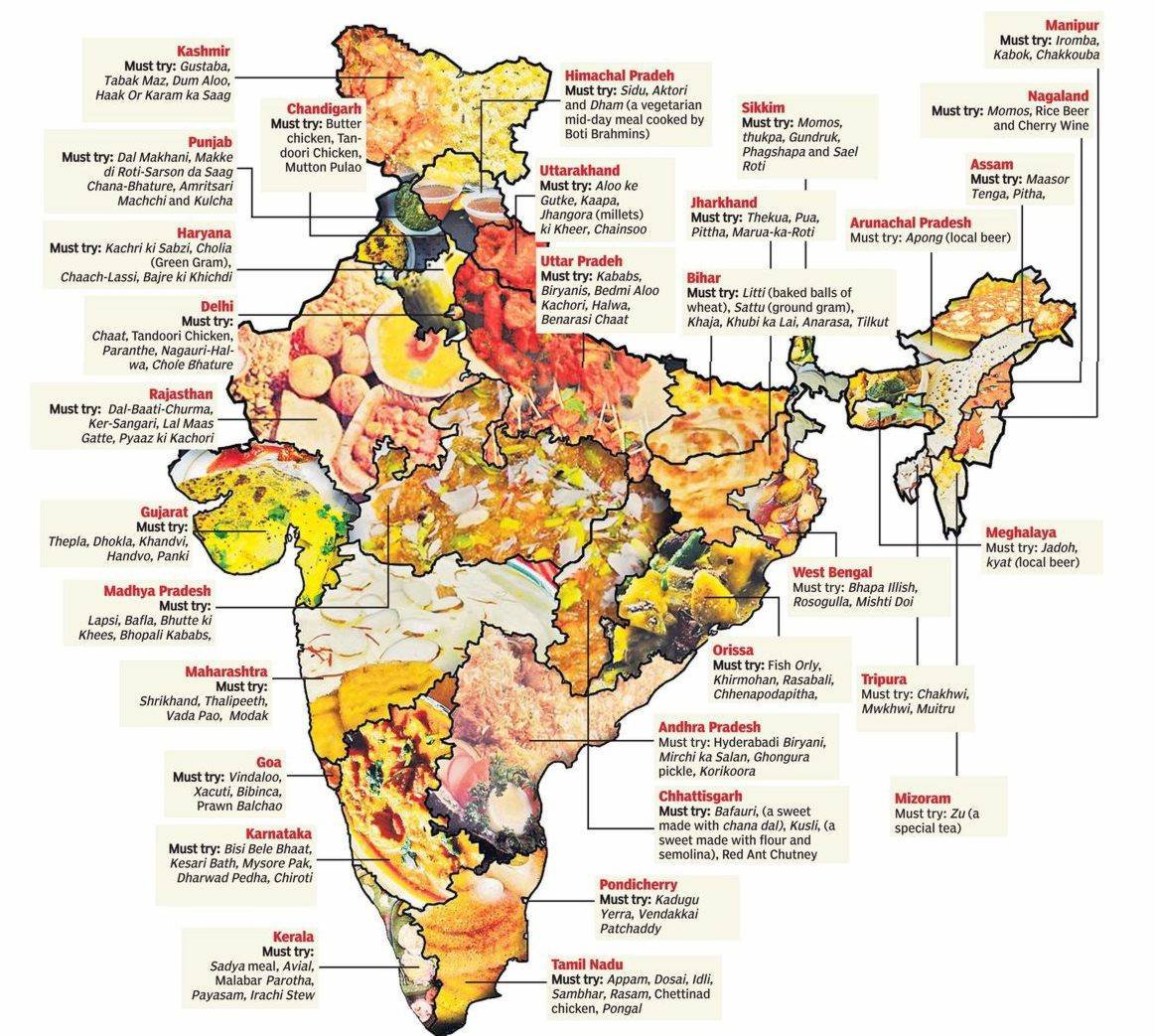This image is an infographic map of India, depicted against a plain white background. The map itself is filled with a variety of colors like red, orange, yellow, and brown to highlight different regions and their renowned cuisines. The map presents regions such as Kashmir, Punjab, Haryana, Delhi, Rajasthan, and Gujarat in red. Each region features small text annotations in black that list iconic foods associated with that area. For instance, in Kashmir, dishes like Gustava, Tuak, Maaz, Dum, Atu, Haak, and Kram Kasang are recommended. Similarly, in Punjab, delicacies such as dal makhani, makh de roti saran de saag, and chana bhatir are highlighted. This pattern of regional specialties continues throughout the map, covering areas like Delhi, Rajasthan, Gujarat, Maharashtra, Goa, and Kerala. Black lines connect each region's name, written in red, to their respective food descriptions, written in black, providing a comprehensive guide to trying local cuisines across diverse parts of India.